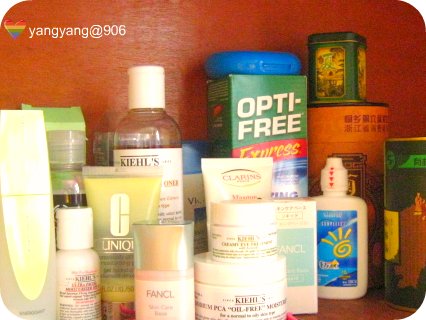A vibrant photograph features a collection of personal care products meticulously arranged on an orange background. At the top of the image, a watermark displays a pride flag heart rendered in shades of red, orange, yellow, green, and blue, accompanied by the name "Yang Yang at 906". The assortment includes a variety of bottles, tubes, and jars in different shapes and sizes. 

Prominently placed is a tall white bottle, standing next to a shorter white bottle that features black and red font. A bottle with a clear lid is positioned in front of a green box. Toward the center, a Clinique package containing a clear fluid with a silver lid catches the eye. Adjacent to these, a short white bottle with a pearlescent lid is visible. 

In the background, a bottle of Kiehl's product, recognized by its white lid, is partially obscured by a white bottle with a blue lid. Next to this, a white jar bearing the Kiehl's logo stacks under another Kiehl’s product, both white. Nearby, a white tube with dark font is positioned behind a white box adorned with a blue label. 

A white bottle with a blue, yellow, and white label, accented by a plastic safety seal marked with red arrows, stands out among the items. A green box with brown elements is paired with an orange container featuring black font. A decorative box in a rich forest green or emerald hue, adorned with a brown and yellow graphic and topped with a green lid, adds to the variety. Finally, a green box labeled "Opti-Free" in white font supports a blue circular object, resting on top.

The careful arrangement and diverse colors of the personal care products create an engaging and aesthetically pleasing visual story against the warm orange background.